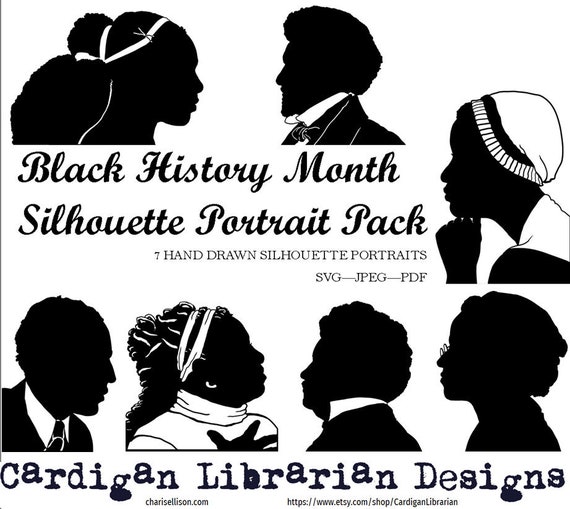The image is a promotional poster for a Black History Month Silhouette Portrait Pack, showcasing hand-drawn silhouettes of various figures. The top of the image features a man and a woman in silhouette, both rendered in black on a white background. Below them, in the center, the text reads, "Black History Month Silhouette Portrait Pack - Seven Hand-Drawn Silhouette Portraits, SVG, JPEG, PDF."

To the right of the main text, there's a silhouette of a woman with a white cap. Below this are several more portraits: a man in a suit with a tie, a woman with her hair pulled back and wearing a white turtleneck and headband, another man in a suit, and another person wearing glasses. All these silhouettes are crafted in a style that evokes the early 19th century, emphasizing simple yet evocative outlines.

At the very bottom, the text "Cardigan Librarian Designs" is visible, along with the URL "https://www.etsy.com/shop/CardiganLibrarian" and the site "KarisEllison.com," highlighting that this is an item available for purchase on Etsy by Cardigan Librarian Designs. The overall theme underscores the historical significance and artistic representation of each silhouette, celebrating Black History Month through these detailed and stylized portraits.